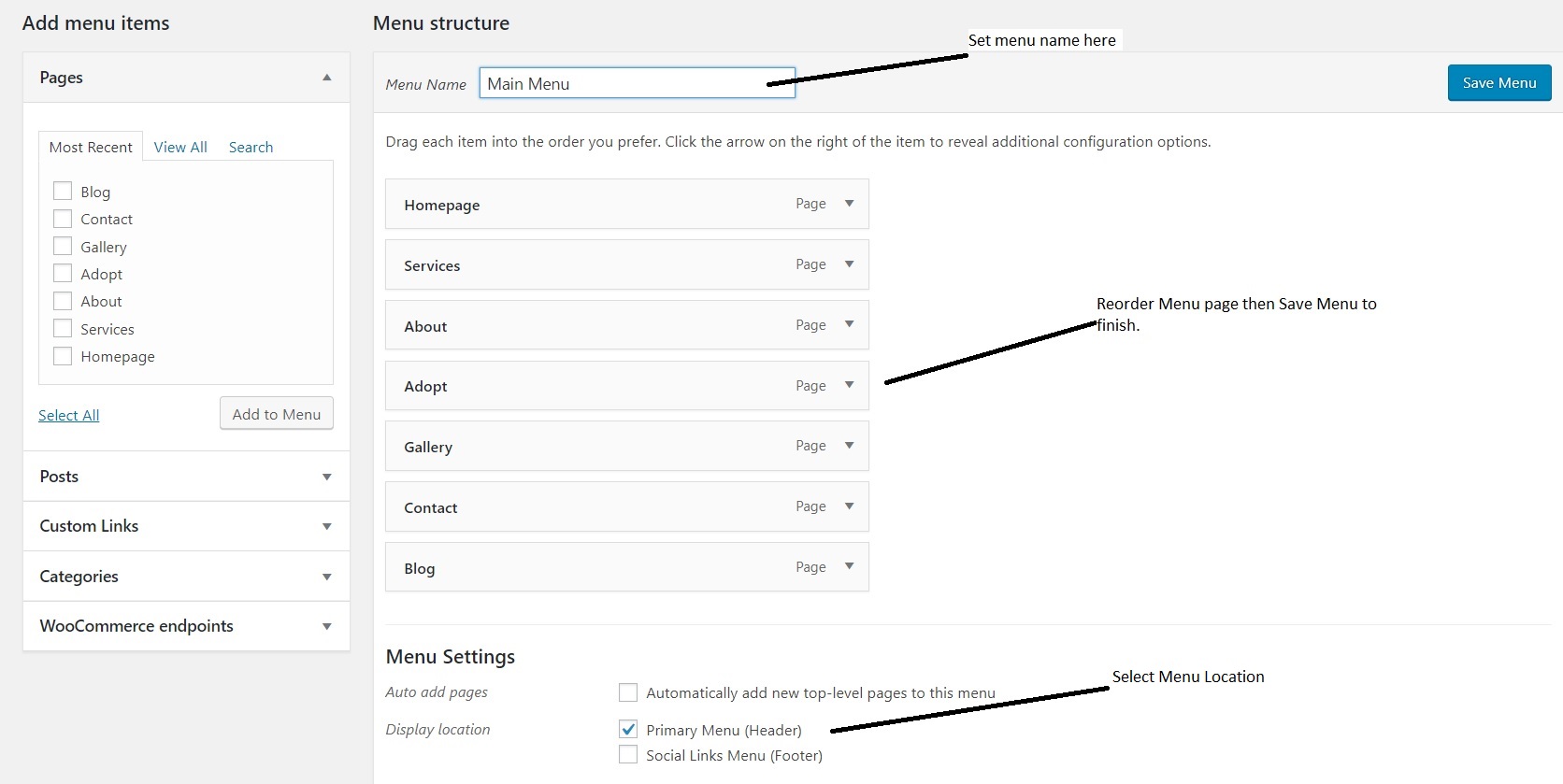The image showcases a user interface for configuring a website menu, divided into two main sections with varying backgrounds. 

On the left side, the section begins with a black background header labeled "Add Menu Items," followed by "Pages." Transitioning to a white background, the interface features three tabs. The first tab, labeled "Most Recent," stands out with black text. Within this tab, there are several checkbox options, characterized by a white fill and black borders. The options listed include: "Blog," "Contact," "Gallery," "Adopt," "About," "Services," and "Homepage." At the bottom of the list, there are additional options labeled "View All" and "Search." Below these checkboxes, there is a gray box containing the text "Add to Menu." To the left of this section, in the tail area, there is a "Select All" option. Further down, in black text, it reads: "Post," "Custom Links," "Categories," "WooCommerce Pinpoints."

On the right side, the section is labeled "Menu Structure," with a menu name field containing "Main Menu," highlighted by a blue outline. A black line connects to the instruction "Set Menu Name Here." Below this, there are instructions to "Drag each item into the order you prefer. Click the arrow on the right for the item to reveal additional configurations." The items listed here include: "Homepage (Page)," "Services (Page)," "About (Page)," "Adopt (Page)." A black line points to "Adopt Page," with the instruction "Reorder Menu, Paste and Save Menu to Finish," followed by "Gallery (Page)," "Contact (Page)," and "Blog (Page)." At the bottom, there are "Menu Settings," which include an option to "Auto-add pages," with a description "Automatically add new top-level pages to this menu." Below this, "Display Location" is checked and labeled "Primary Menu Header." Another black line connects this to the instruction "Select Menu Location." The final option is labeled "Social Links Menu" with a note in parentheses indicating it is for a specific purpose or number.

This detailed caption captures the intricate layout and specific elements of the user interface for configuring a website menu.